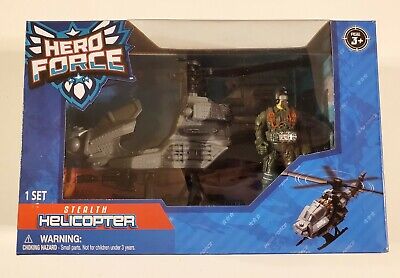This image features a vividly detailed package containing a child's toy set, prominently showcasing a stealth helicopter and an action figure. The background of the vintage-style poster is blue, with a distinct bright red stripe on the left side displaying the words "Stealth Helicopter" in block font. A warning sign stating "Choking Hazard" is situated just below the stripe, cautioning that the toy is suitable for children aged 3 and above, as indicated by the age recommendation in a black circle with white text in the upper right corner. The upper left corner features the logo "Hero Force" in a bold white, blue, and black superhero font style.

The lower right corner of the poster is adorned with artistic imagery of the gray helicopter, emphasizing its sleek design. The toy set itself is displayed within a clear plastic window, part of a cardboard box, allowing for a clear view of the contents. Inside, the action figure, clad in a green combat outfit with a red accessory that seems like a diving jacket, stands separately from the gray and black helicopter. This presentation sparks imaginative play, inviting children to place the figurine inside the helicopter and engage in heroic adventures. The phrase "One Set" confirms the package includes both the action figure and the helicopter.